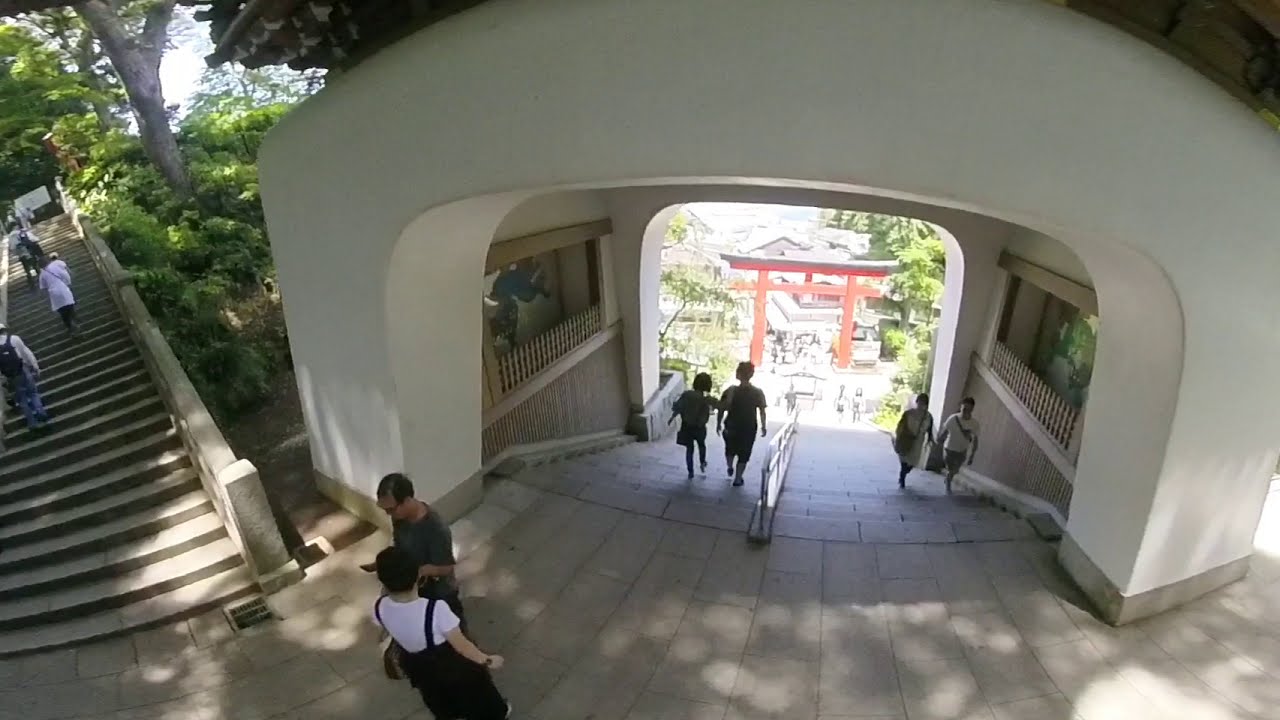The image, likely captured by a security camera during daytime, showcases a bustling scene of approximately 20-30 people, predominantly Asian, moving along a large white staircase and through a smooth white concrete archway towards a distant temple. The staircase, divided by a central metal handrail, sees a few individuals in motion; notably, a couple in black descending, and another in white, holding hands, ascending the right side. The bright, sunny atmosphere illuminates the greenery, shrubs, and a myriad of trees in the background, emphasizing the verdant landscape. A significant, ornate, orange wooden structure, suggestive of a Japanese temple or garden gateway, stands prominently at the bottom. In the foreground, a man in glasses and a gray shirt is observed looking down, accompanied by a woman in a black jumpsuit and white T-shirt. The dynamics of the scene imply a mix of locals and tourists, given the presence of bags and cameras among the crowd.